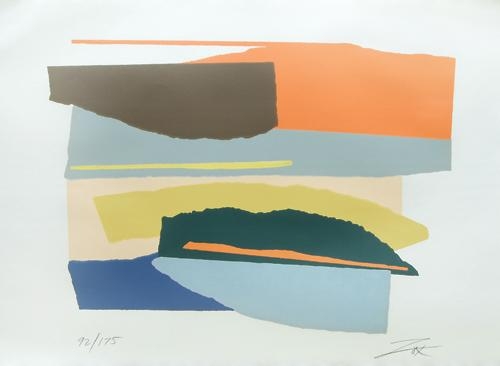This image showcases an abstract, postmodern painting on a very light pale blue background. The artwork features a central eclectic design composed of numerous torn and layered shapes that appear to be fragments of construction paper, each in various colors including light blue, orange, brown, blue, yellow, green, dark blue, gray, and peach. The design is abstract and disordered, resembling chips or flecks of materials pasted together to form a visually striking collage.

Starting from the bottom left, we have a blue rectangle overlapping with a lighter blue torn piece. Above these, there's a green piece intersected horizontally by an orange stripe, resting just above a mustard yellow strip. Further up, a piece of light peach-colored paper is overlaid with another thin blue strip, which itself is adorned with a yellow stripe extending from the center to the left edge. A thick, ripped piece of brown paper sits prominently next to a fragment of orange paper on the right.

Towards the bottom left corner, the notation "92/175" is handwritten, which likely indicates the artwork’s edition number. Just above the bottom right corner, there’s a signature that appears to read "ZOX," with the Z being notably large. This text corroborates the individuality and originality of the artisan's creation. This piece epitomizes a low-quality artwork, possibly part of a personal portfolio rather than a polished gallery piece, yet it exudes a unique charm and intricate detail that beckons a closer inspection.